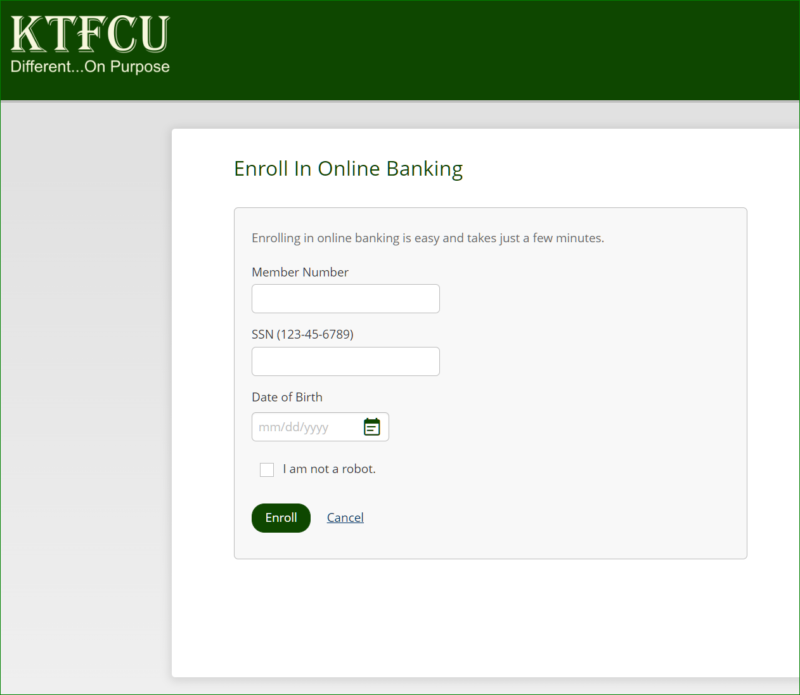The image depicts a user interface from an online banking platform, specifically from a bank identified as KTFC. The screen is a step-by-step form for enrolling in online banking services. At the top, a straightforward message reads, "Enrolling in online banking is easy and takes a few minutes."

The form consists of several fields requiring user input. These include:

1. **Member Number**: A text box for entering the user's member number.
2. **Social Security Number**: A text box for entering the user's Social Security Number.
3. **Date of Birth**: A text box accompanied by a calendar icon for selecting the user's date of birth in the specified format.

Additionally, there is a reCAPTCHA checkbox labeled "I am not a robot" to verify that the user is human.

At the bottom of the form, there are two buttons: a prominent green button labeled "Enroll" for submitting the form and a cancel button for aborting the process.

The layout is simple and user-friendly, indicating a streamlined process for existing bank members to access online banking features conveniently from their devices.